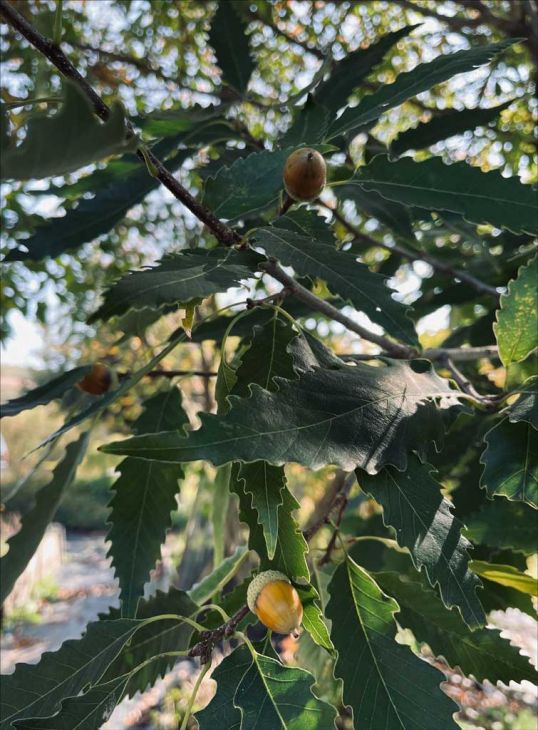This image is an extremely close-up digital photograph of hickory nuts growing on a tree, surrounded by dark, deep green leaves with jagged edges that come to a point. The photograph captures two almost ripe hickory nuts, which are tan in color and still encased in a lightly covering husk. At the top view, one can observe the characteristic pointy protrusion of the hickory nuts, resembling a thistle. The green leaves contrast sharply with the light beige, almost round or oval-shaped nuts. Additionally, the nuts feature small caps on their tops, which are slightly different in color than the nut itself. The background of the image shows light filtering through, illuminating parts of the composition and contributing to the detailed textures of the foliage and the nuts. There are elements such as vines, branches, and rocks present, adding to the natural setting of the scene.